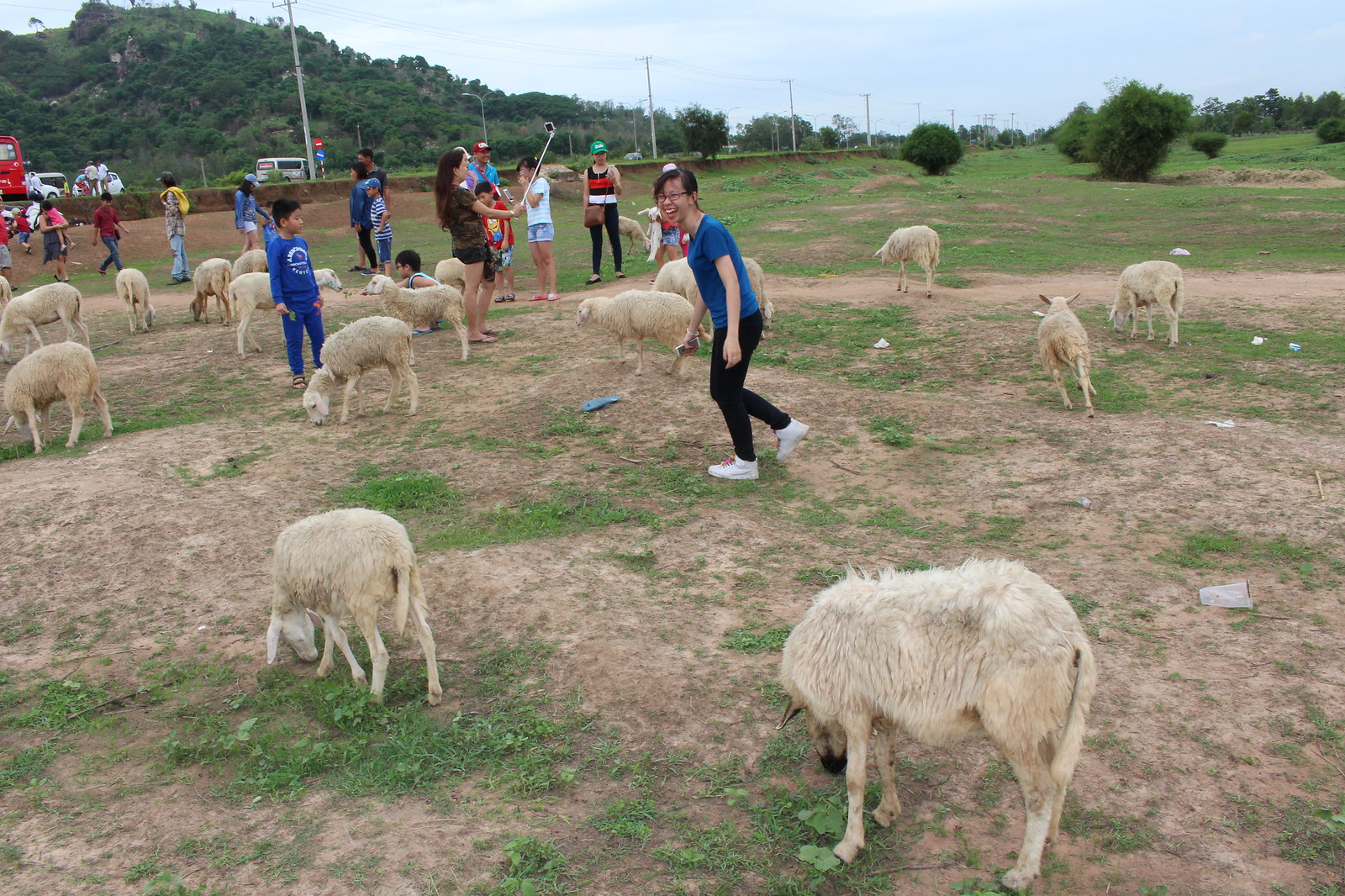This horizontal outdoor photograph captures a lively scene in a large field, where the ground consists of sparse, patchy grass and dry, compacted dirt. The upper portion of the image features a blue sky with white clouds, a forested hill in the upper left corner, and telephone wires extending toward the right. The background includes green bushes, trees, a road with a retaining wall, light poles, and several vehicles, with people standing and conversing.

In the foreground and middle ground, a group of cream-colored animals—likely recently shorn sheep, although possibly goats—are scattered around, mostly with their heads down, grazing on the sparse grass and hay. The animals appear skinny and light-colored, each with tails and four legs.

Among the animals, numerous people, including men, women, and children, are interacting. The focal point is a woman in the center, wearing a blue short-sleeved shirt, black pants, and white sneakers. She is mid-step, smiling broadly, and appears to be laughing. To her left, a boy in a blue sweatsuit stands near one of the animals.

In the background, a girl holding a selfie stick captures the moment, emphasizing the social nature of the gathering. Another individual, possibly a girl, wields a long blue object, potentially a golf putter. The scene is vibrant with human and animal interaction, set against the contrasting backdrops of natural and man-made elements.